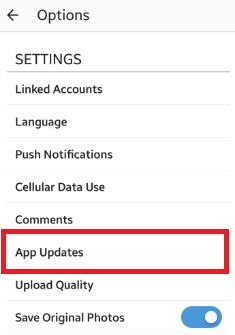This image is a vertical screenshot, likely taken from a mobile device, with a minimalist white background and no borders. At the top of the image, there is a grayish header labeled "OPTIONS" with a left-pointing arrow next to it. Directly beneath the header, "SETTINGS" is prominently displayed in uppercase letters. Following this are several menu items each listed on their own line: "Linked Accounts," "Language," "Push Notifications," "Cellular Data Use," "Comments," and "App Updates." "App Updates" is highlighted with a bold red rectangle, indicating it has been selected. Below "App Updates," the menu continues with "Upload Quality" and "Save Original Photos." To the right of "Save Original Photos," there is a blue oval switch, which is turned on, indicating the option is enabled. The screenshot is straightforward, focusing solely on the settings menu without any additional elements or distractions.